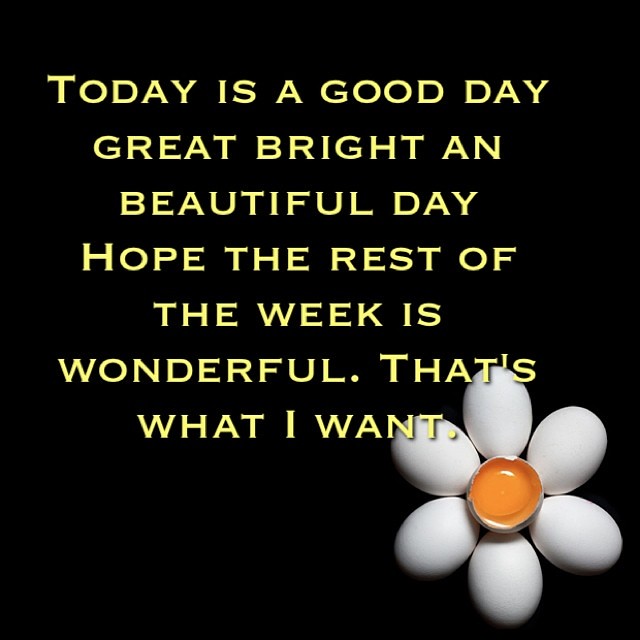The image features a predominantly black square background with vibrant yellow text taking up most of the space. The text, written in large, bold capital letters, reads: "Today is a good day. Great, bright, and beautiful day. Hope the rest of the week is wonderful. That's what I want." Notably, there is a minor grammatical error in the second line—it should read "and a beautiful day." 

In the lower right-hand corner, there's a unique and eye-catching element: a configuration of six white eggs arranged in a circular pattern surrounding a half-cracked eggshell that reveals the yellow yolk inside. This arrangement resembles a flower, with the intact eggs forming the 'petals' and the yolk representing the 'center' of the blossom, evoking the look of a sunflower or carnation. This intriguing composition could suggest a greeting or positive message, adding a whimsical touch to the motivational quote above.